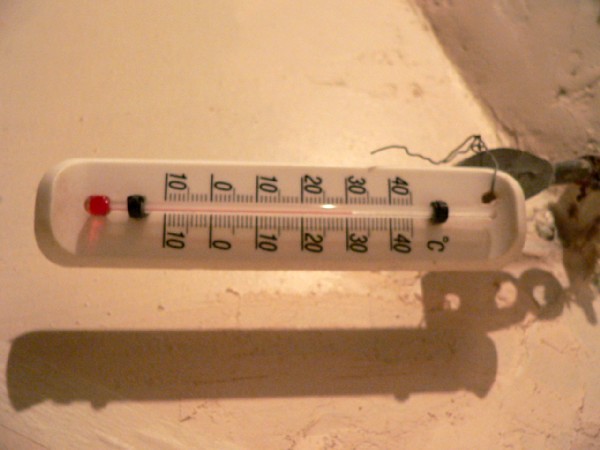On a light pink concrete background, both the wall and the surface exhibit a uniform texture. Centrally, a dark spot punctuates the concrete, surrounded by a piece of black rubber pipe and a small protruding rock. Nearby, a white thermometer lies horizontally, secured to the concrete by a wire. The thermometer features dual measurements, with Celsius markings on the right and Fahrenheit on the left, and visible mercury at the bottom of the bulb. It is mounted on a small plastic board with rounded ends, held in place by two black clips.